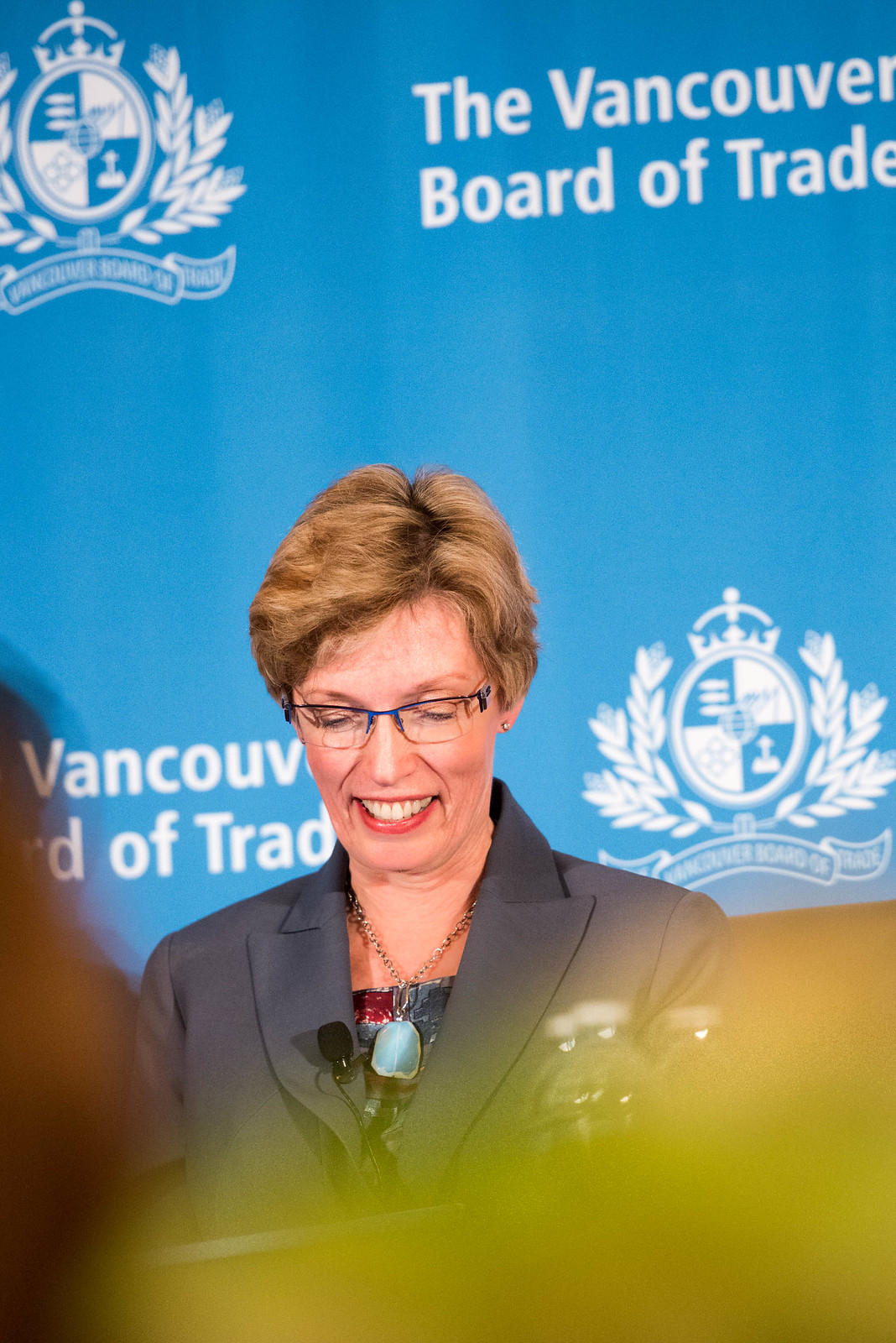The image depicts a middle-aged woman, likely in her 50s or 60s, standing on a stage against a light blue background that prominently features the text "Vancouver Board of Trade" in both the upper right and lower left corners. She is positioned in the center lower half of the image, dressed professionally in a dark gray suit over a red, blue, and square-patterned shirt. A necklace with a large light blue medallion hangs around her neck. The woman has short, light brown hair with visible roots, wears square-shaped glasses with blue rims, and has a black microphone clipped to her lapel. She appears to be looking down, perhaps reading or speaking to an audience, and is smiling slightly. The background also includes white symbols resembling a seal or shield with a crown and oak leaves, positioned in the upper left and lower right corners. In the foreground, near her left shoulder, there are three water bottles. The bottom of the image is partly obscured by out-of-focus objects, including a large yellow blur and a darker shape on the left side.